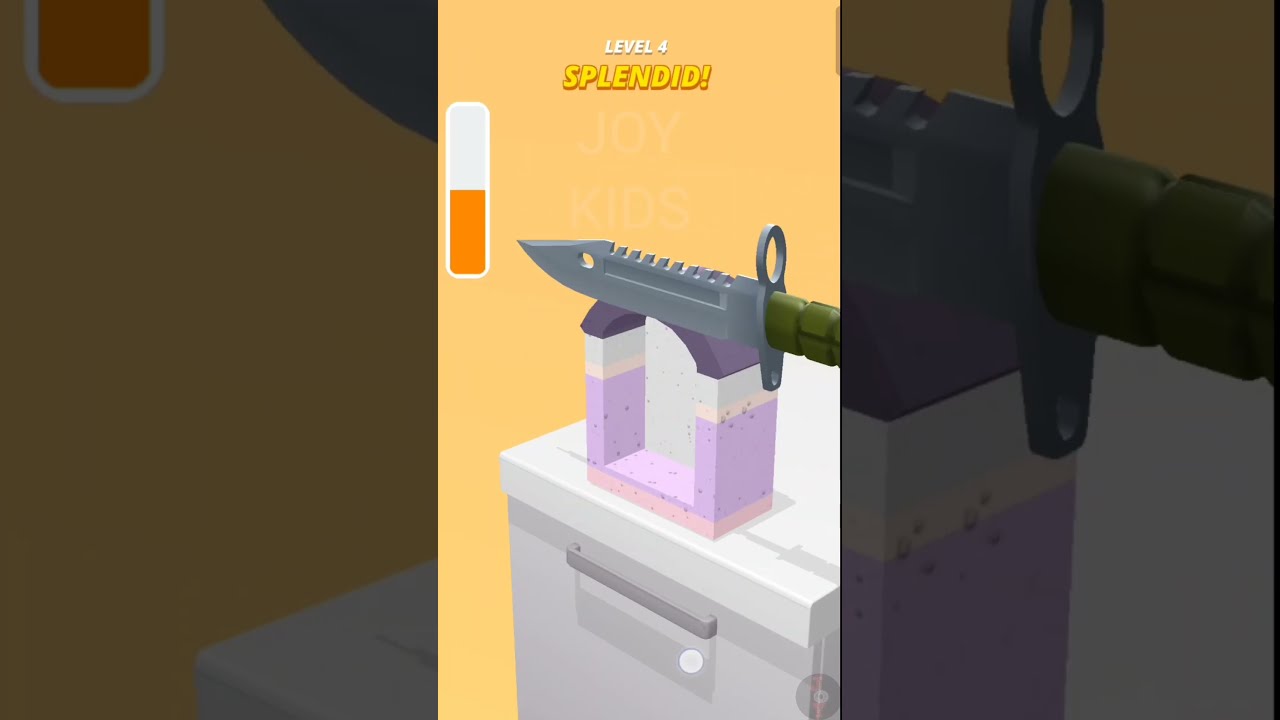The central image showcases a still from a video game or app, prominently featuring a white cabinet or table with a purple arch-like object on top. Sitting atop this arch is a large hunting knife with a silver blade and a green handle, creating a striking and somewhat out-of-place visual. Above this scene, in the middle-top portion of the image, the text "Level 4" appears in white, followed by "Splendid" in large yellow all-caps. The entire image has a light orange background, which is further replicated, darkened, and zoomed in to fill the vertical sides surrounding the central picture. On the left side, there's a vertical bar, half orange and half white, enhancing the intricate layout and design of the game's interface.